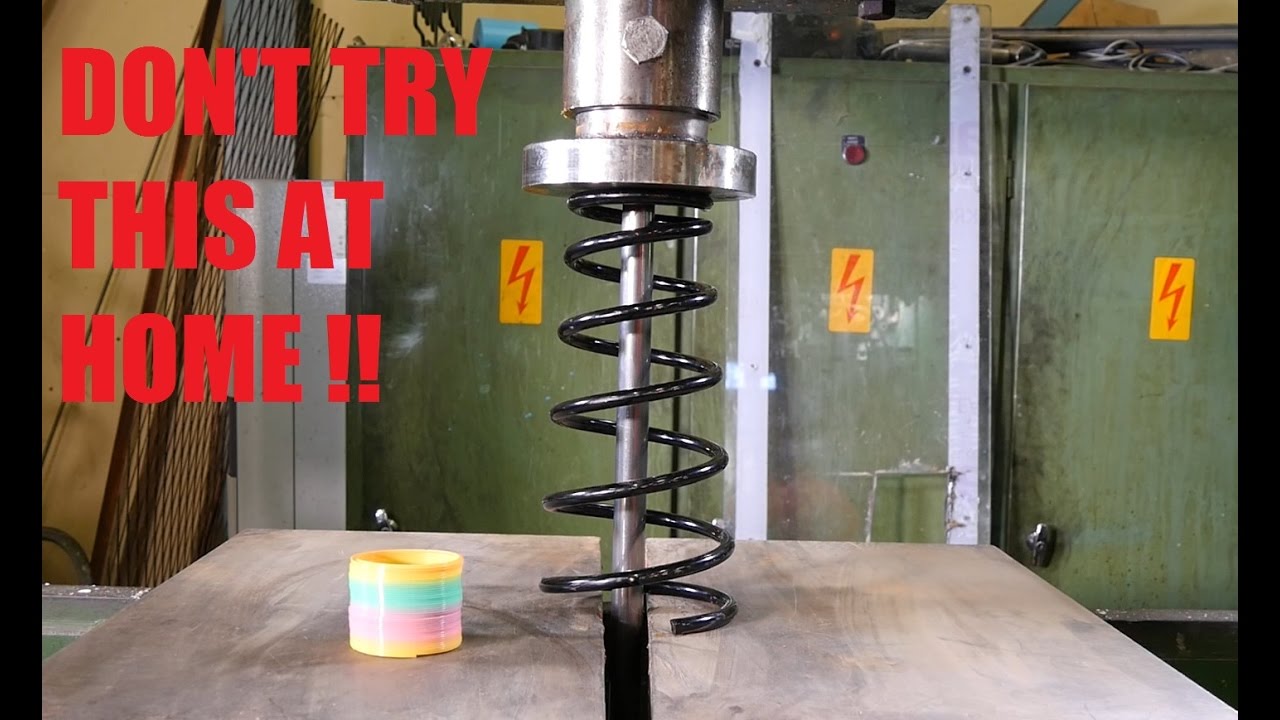In a workshop-like setting, an image features prominent red text in the upper left corner that warns "DON'T TRY THIS AT HOME!!" Various green cupboards, each adorned with yellow signs displaying red electric symbols, line the yellowish wall in the background. The cupboards also have red, but currently turned-off, indicator lights. To the left, a piece of a gate leans against the wall. In the foreground, a wooden table holds a central metal drill-like device, featuring a thick round top and a black coil winding around its metal bar. Nearby, a yellow roll and lines of blue and pink string or coils, resembling a multicolored slinky, are scattered across the table.